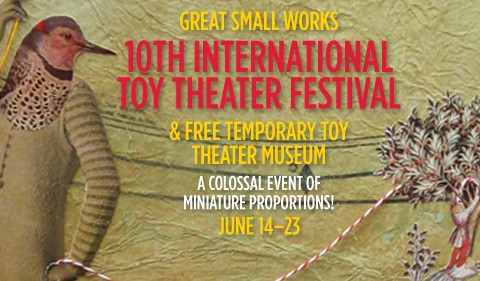The advertisement poster for the Great Small Works 10th International Toy Theater Festival and Free Temporary Toy Theater Museum, running from June 14th through the 23rd, is set against a textured, light green background reminiscent of wrinkled parchment paper. The top of the poster reads "Great Small Works" in bold yellow letters, followed by "10th International Toy Theater Festival" in prominent red text. Below that, in smaller yellow text, it announces the "Free Temporary Toy Theater Museum" and describes the event as "A Colossal Event of Miniature Proportions" in white letters. The date, "June 14th through the 23rd," is also highlighted in yellow.

The artistic depiction on the left side of the poster features a whimsical figure with the head and partial body of a bird, dressed in a green outfit with a darker green striped sleeve. This bird-human hybrid is theatrically posed, holding a white and red rope that extends across the poster to a tree where another person is seen tying the rope around the trunk. The image, abstract and artful, adds a surreal touch to the design, enhancing the intriguing allure of the festival and museum event.